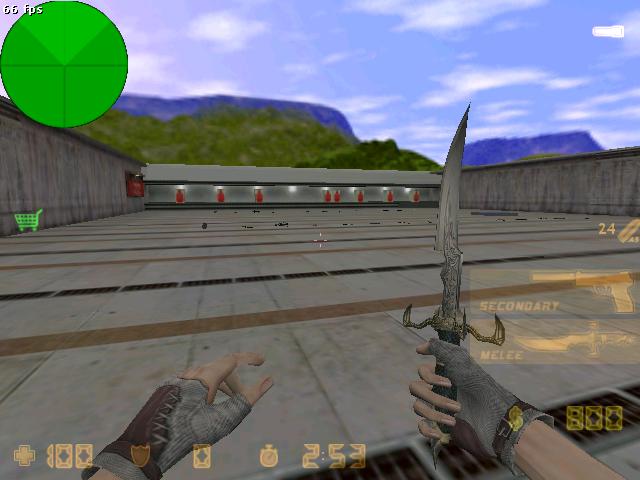This image is a screenshot from a video game, depicting a first-person perspective where only the character's hands are visible. The character wears fingerless gloves combining grayish cloth and brown leather with visible stitches. The left hand is empty while the right hand holds an intricate dagger with elaborate designs and a yellowish hilt. The setting appears to be some sort of training or battle arena, characterized by a large, flat, gray surface with brown and black stripes forming a grid-like pattern. Red, human-shaped target outlines are seen on a shorter wall at the far end, with white light-like areas above their heads. 

The background features green rolling hills, blue mountains, and a sky filled with clouds. In the top left corner of the screen, UI elements include a green mini-map circle, a green shopping cart icon, and several statistics showing a frame rate of 66 FPS. Below this, yellow indicators display a shield icon and a value of 100, plus additional game stats for a secondary weapon, a melee knife icon, and a currency symbol with a value of 800. On the right, an orange translucent box lists a timer set at 253 seconds and icons representing different weapons.